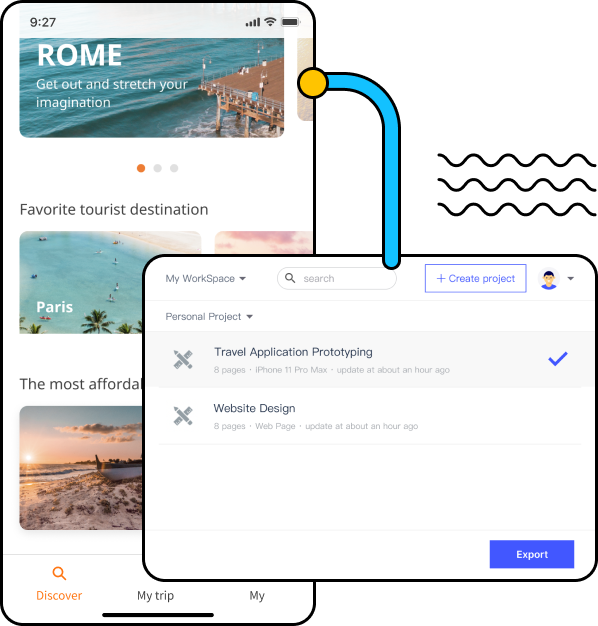In this image, we see a detailed interface that appears to be part of an advertisement blended with a project management or design application. 

Near the lower center, a black-outlined rectangle prominently features the label "My Workspace" with a drop-down arrow beside it. To the right of this label, there is a search bar for querying the workspace contents. 

In the upper right-hand corner of the interface, the phrase "Create Project" is written next to a plus symbol, indicating a button for adding new projects. Adjacent to this, there is a small profile icon, suggesting user account options.

Below the main workspace label, the text "Personal Project" is displayed, followed by a list of projects. "Travel Application Prototyping" is highlighted, indicating it is currently selected. Beneath this, another project title reads "Website Design." 

In the bottom right corner of this rectangle, a button labeled "Export" is visible, likely intended for exporting project data.

In the background, partly obscured by the foreground elements, a larger black-outlined rectangular area is visible. At the top of this background section, an image with the text "Roam, Get Out, and Stretch Your Imagination" is displayed, promoting adventurous travel. Underneath, the words "Favorite Tourist Destination" are written, with a visible photo of Paris. Further down, the phrase "The Most Affordable" appears but is partially covered by the overlaying project interface.

At the very bottom of this background area, three navigation buttons are visible, labeled "Discover," "My Trip," and "My" in the bottom right corner. These buttons likely serve as options for navigating different sections of the application.